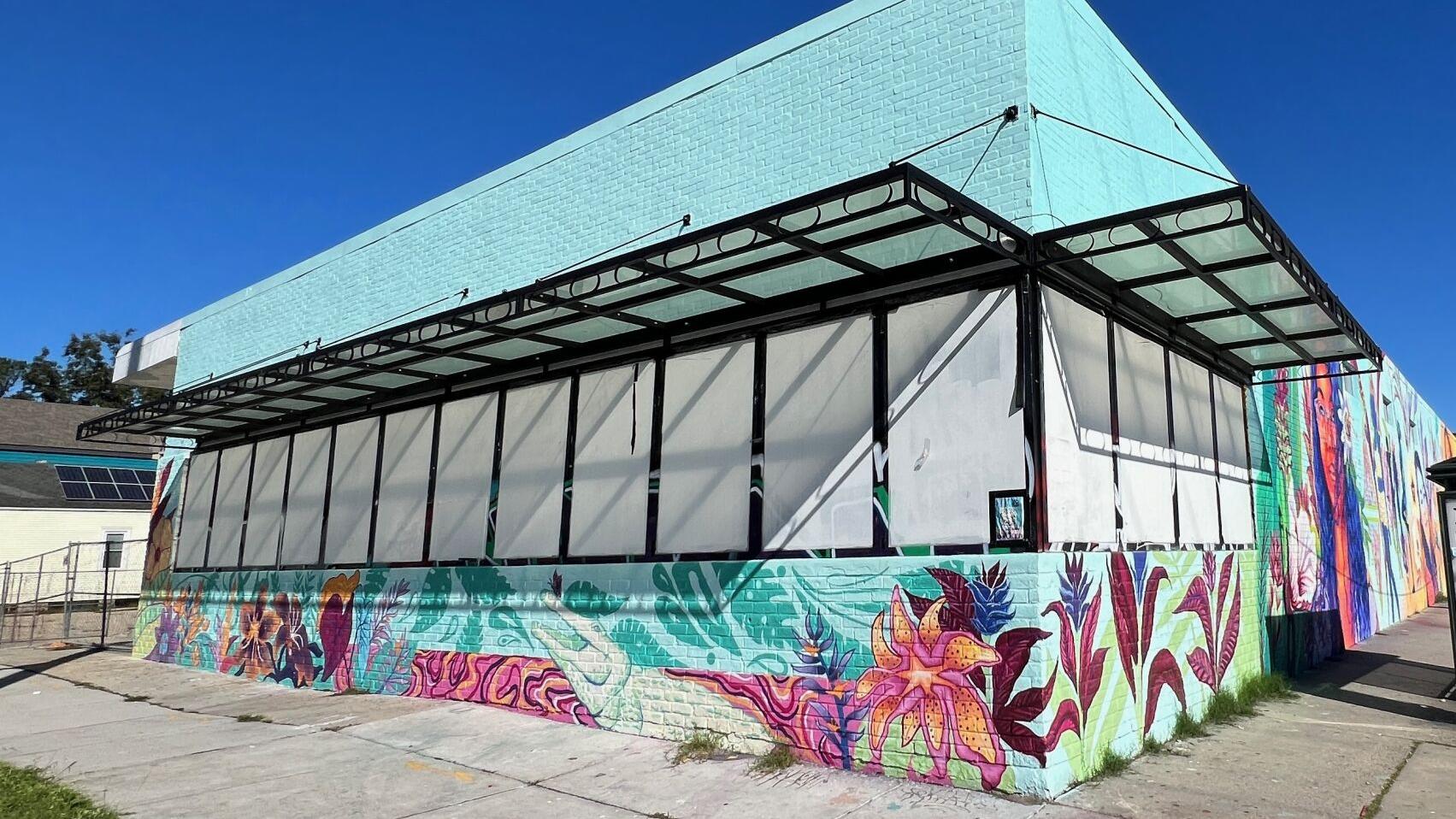The image depicts a small building set against a vibrant blue sky on a bright, sunny day, likely during spring or summer, as indicated by the leafy trees in the background. The building is predominantly painted in a light turquoise or teal color, contributing to its lively appearance. The lower half of the building showcases a cheerful and brightly colored mural featuring a variety of flowers, including big yellow blossoms and plants with maroon leaves, as well as an image of a woman with long, dark hair. The mural extends to a long wall on the right, which is adorned with street art and additional colorful designs. A wide row of windows runs along the middle of the building on both sides, though they are obscured by white paper, hinting that the building may no longer be in use. The front windows have what seem to be non-functional lights hanging above them. Surrounding the building is a concrete sidewalk, and to the left, a fence is visible. The top of the building remains unpainted, adding a light blue or aqua hue to the overall aesthetic. In the distant background, another building appears, possibly equipped with solar panels.